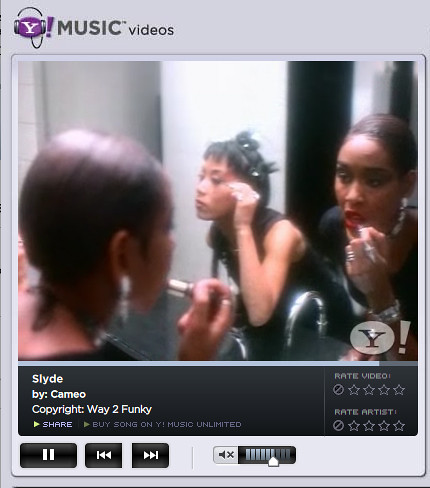The image is a screenshot from an old Yahoo Music video player interface. At the top, the Yahoo Music logo is prominently displayed with a distinctive purple "Y" encircled and wearing headphones, accompanied by the word "MUSIC" in bold black uppercase text, with "videos" written in smaller text beneath it. The main content features a mirror reflection of two Black women applying makeup. The woman on the left, seen only in the mirror, has darker black hair and is adjusting her eye makeup with her hand. The woman on the right, also visible directly and in the mirror, has brown hair and is applying lipstick. She is dressed in black with a white necklace. Below the image, the text reads "SLYDE dances by Cameo," followed by the copyright notice, "Way Too Funky." On the right side of the interface, there is a small green triangle icon for sharing. Additionally, there are buttons for rating the video and the artist, as well as playback controls including pause, fast forward, rewind, and volume adjustment sliders.